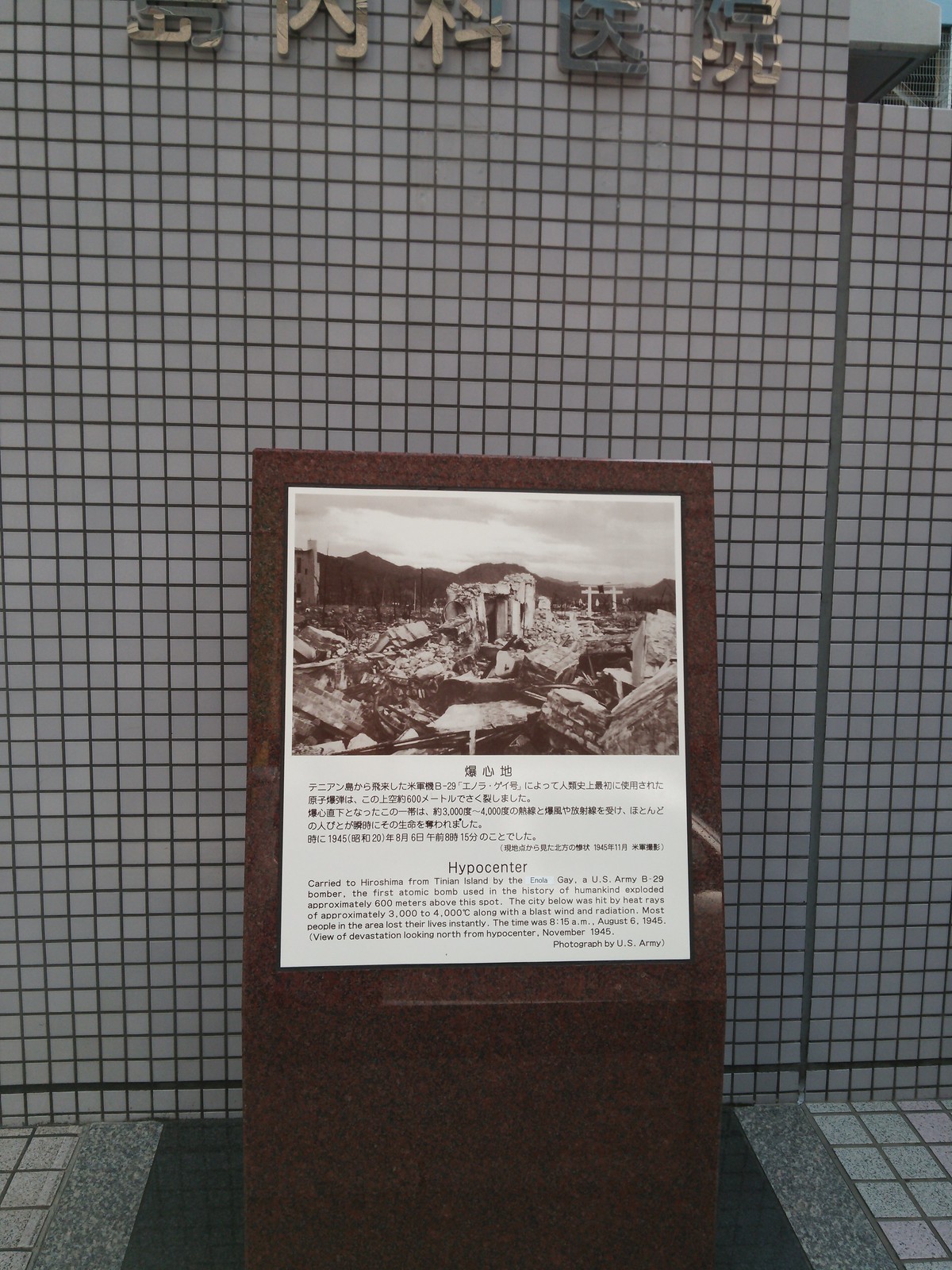The image depicts a memorial display situated on a green-carpeted area between a tiled floor and a display shelf. The primary structure is a brown-colored display shelf, possibly made from wood or stone, set against a backdrop of a gray-tiled wall with black square accents. At the top of this wall, large Chinese characters are prominently affixed, suggesting the importance or name of the memorial. 

On the display shelf, there is a plaque with a photograph at the top depicting extensive devastation, including crumpled buildings and scattered debris. Notably, two white crosses can be seen in the right portion of the photograph, which adds a poignant touch to the scene of destruction. Below the photograph, text in Japanese characters offers further explanation, with an accompanying English translation providing historical context. 

The English text reads: "Hypocenter. Carried to Hiroshima from Tinian Island by the Enola Gay, US Army B-29 bomber, the first atomic bomb used in the history of humankind exploded approximately 600 meters above this spot. The city below was hit by heat rays of approximately 3,000 to 4,000 degrees centigrade, along with a blast wind and radiation, causing most people in the area to lose their lives instantly. The time was 8:15 a.m., August 6, 1945." A footnote indicates that the photograph was taken by the US Army and describes the view of the devastation looking north from the hypocenter in November 1945.